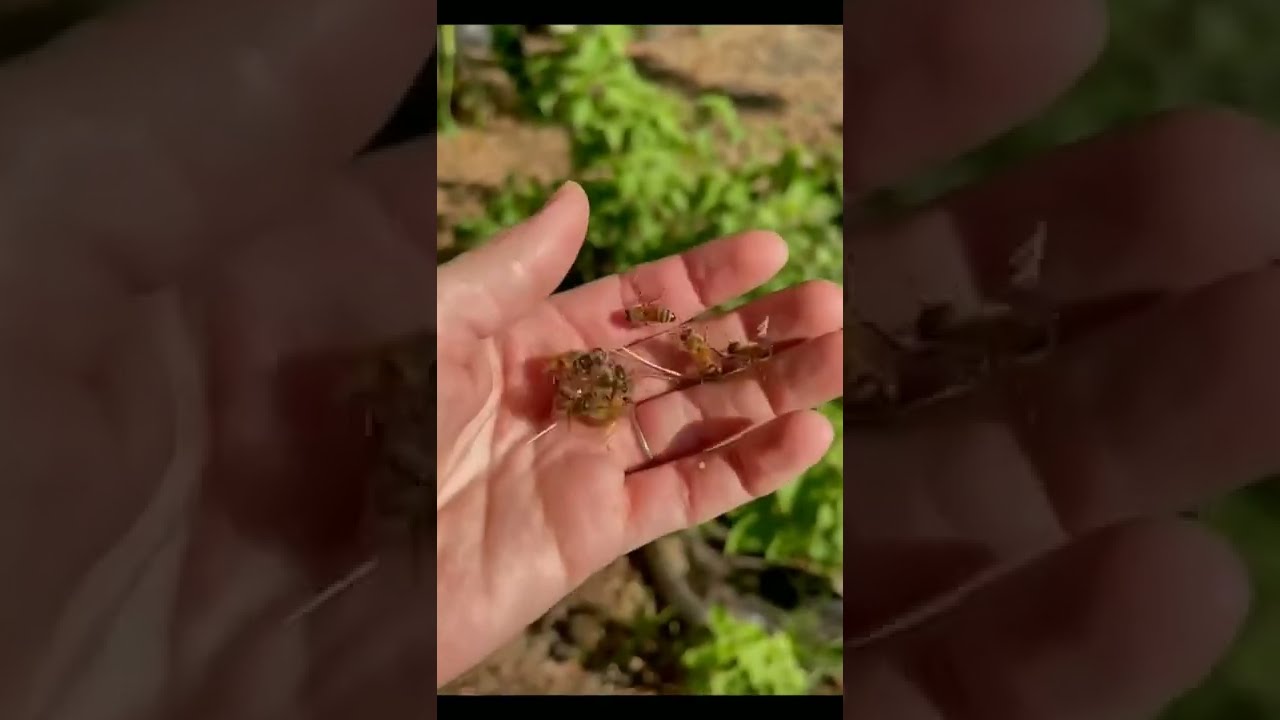The image appears to be an outdoor shot, possibly intended as a thumbnail for a TikTok or social media video. The focal point is an open hand, belonging to a person who might be a white man or woman, adorned with a ring. The hand is holding a cluster of bees, snugly huddled together in the center of the palm, with a few more bees scattered around. The background, although slightly blurry, displays a vibrant green landscape with vegetation. There's a hint of a green leafy plant or tree in the backdrop, possibly a marijuana plant, amidst the brown, sandy ground. The entire image is framed with a black or grayed-out border, enhancing the central subject. The setting gives the impression of a farm, perhaps where the person is interacting with bees, possibly collecting honey.